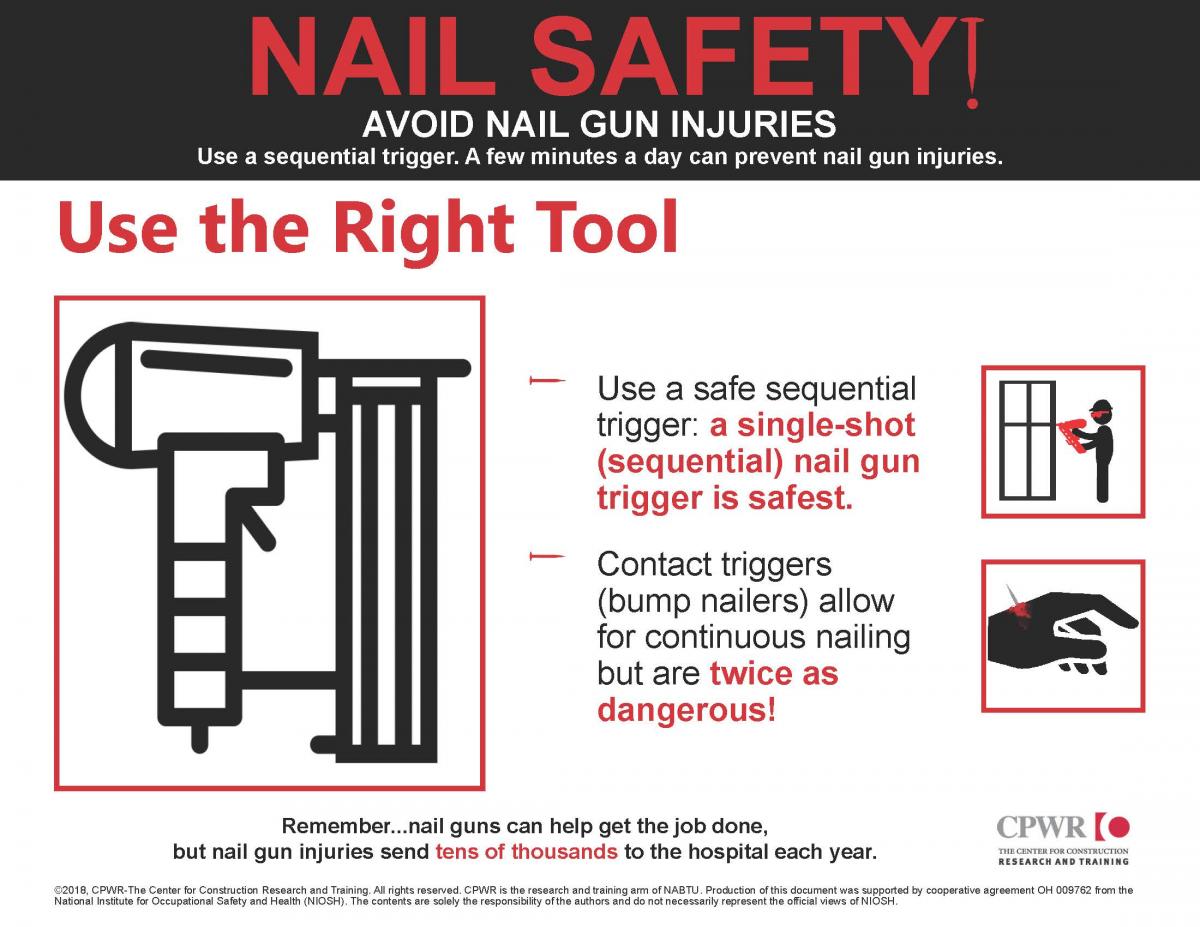This image is a detailed safety advertisement designed for builders and carpenters, emphasizing the importance of using sequential triggers on nail guns to prevent injuries. The advertisement is in landscape orientation and predominantly features black-and-white illustrations with spot color accents in red. 

At the top of the poster is a bold black horizontal banner with the main headline in red and white text: "NAIL SAFETY!" followed by a cautionary message in smaller white text: "Avoid nail gun injuries. Use a sequential trigger. A few minutes a day can prevent nail gun injuries."

The main body of the poster has a white background with red text and multiple illustrations. On the top left, red text reads, "USE THE RIGHT TOOL!" accompanied by a black-and-white line drawing of a nail gun bordered in red. Adjacent to this illustration, bullet points provide further safety instructions. 

To the right, there are two smaller red-bordered square illustrations: the top square shows a man wearing safety glasses using a nail gun near a window, and the one below depicts a hand with a nail piercing through it, causing visible bleeding. 

Between these illustrations, the text advises: "Use a safe sequential trigger. A single shot nail gun trigger is safest. Contact triggers allow for continuous nailing but are twice as dangerous."

At the bottom of the poster, more text emphasizes: "REMEMBER NAIL GUNS CAN HELP GET THE JOB DONE, but nail gun injuries send tens of thousands to the hospital each year." The bottom right corner features the logo "CPWR" with the words "Research and Training" underneath.

This visually striking and informative advertisement aims to promote safer nail gun practices to reduce the risk of injuries.